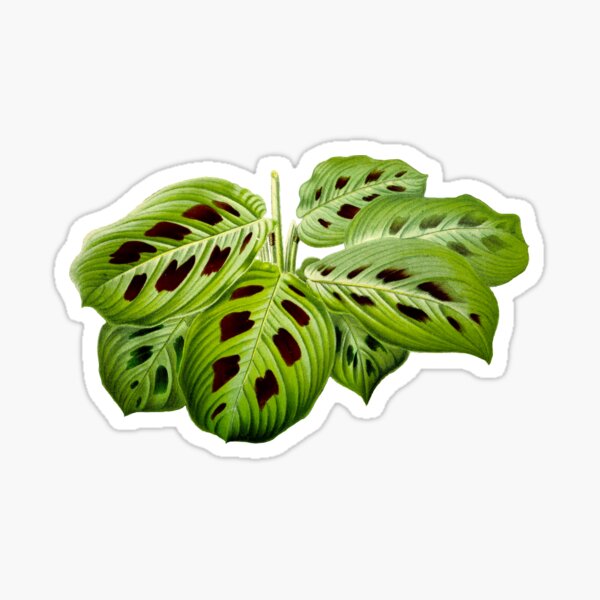The image depicts a sticker featuring seven broad, flat, and ribbed green leaves adorned with multiple dark brown splotches that resemble the spots found on a ladybug. These splotches are scattered across the surface of the leaves, potentially indicating disease, insect damage, or a natural characteristic of the plant species. The leaves are arranged in a bunch with visible stems, and the sticker itself is cut into the shape of these hosta-like leaves. The entire sticker is bordered in white, creating a sharp contrast with the light cream-colored background upon which it is set, giving it a clearly defined edge suitable for display or sale.